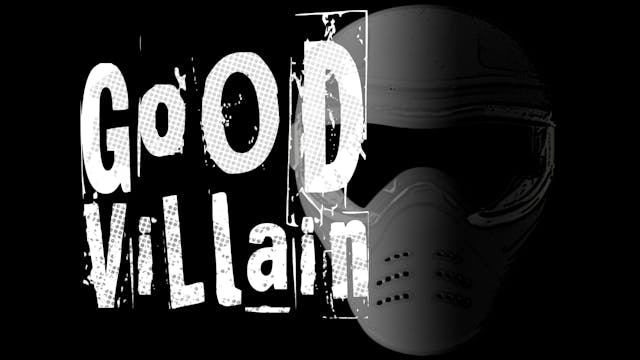The image features a stark, black background with a prominently placed, masked figure on the right side. The mask, which resembles either a hockey or ski mask, is mostly gray and partially shrouded in shadow, making it difficult to discern fine details on the right side. The left side of the mask is more visible, displaying eye holes and a series of breath holes arranged in three vertical sets. Overlaid on the left side of the image is the text "GOOD VILLAIN," with "GOOD" stacked above "VILLAIN." The letters are white with a sporadic gray checkerboard pattern, and the text is rendered in an ominous, ransom-note-like font. The word "VILLAIN" fades out towards the right, adding to the eerie atmosphere of the image.